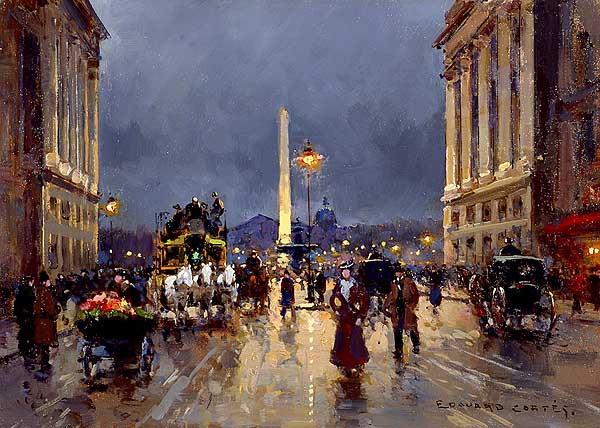This detailed oil painting by Edouard Cortes depicts a vibrant Parisian boulevard scene, likely set in the late 19th or early 20th century. The wide street is bustling with life, as elegantly dressed men and women stroll along, their attire reflective of the period, reminiscent of the late Victorian or early Edwardian era. Central to the composition is a woman in the foreground, wearing a brown coat that extends from her shoulders down to her ankles. The boulevard is flanked by tall, imposing buildings on both sides, showcasing grand architectural features. 

To the left, a flower seller is captured, offering bright red flowers. In the heart of the scene, there is a well-lit monument or long tower, adding a focal point to the busy street. A large lamp post stands prominently next to this monument, illuminating the nighttime ambience. In the background, a white arch rises, with a fountain in front of it, creating a scenic backdrop. Beyond the arch, hills and a night sky contribute to the depth and atmosphere of the painting.

Horses and vintage cars add to the historical charm of the setting. Despite the bustling activity, there is an element of tranquility, enhanced by the foggy air, which gives the painting a certain nostalgic feel, very much like scenes from Mary Poppins or early 20th-century London streets. The artist's signature, Edouard Cortes, is subtly placed in the lower right corner, confirming the painting's authenticity and period charm.